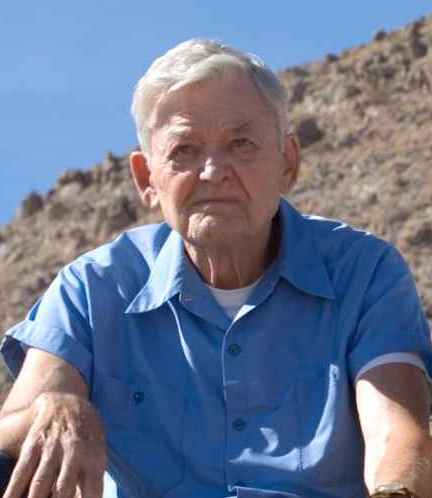The photograph captures a detailed and realistic portrait of the elderly actor, Hal Holbrook, from the top of his head to his upper stomach. Holbrook is dressed in a light blue, short-sleeve button-up shirt with blue buttons, the top button intentionally unbuttoned, revealing a short sleeve white undershirt beneath. The shirt features pockets on both sides of the chest, each secured by a blue button. His gray and white hair is neatly combed to the side, complementing his weathered yet distinguished look. Holbrook's facial expression is a mix of solemnity and introspection, with a subtle half-smile and visible wrinkles adding character to his face. His arms rest partially visible by his sides, with his right hand slightly raised towards the bottom left corner of the image, suggesting motion or a gentle gesture. The background depicts a barren rocky hillside characterized by tan rocks and brown dirt, typical of a southwestern landscape, under a clear, light blue, cloudless sky, indicating that the photograph was taken outdoors in the daytime.